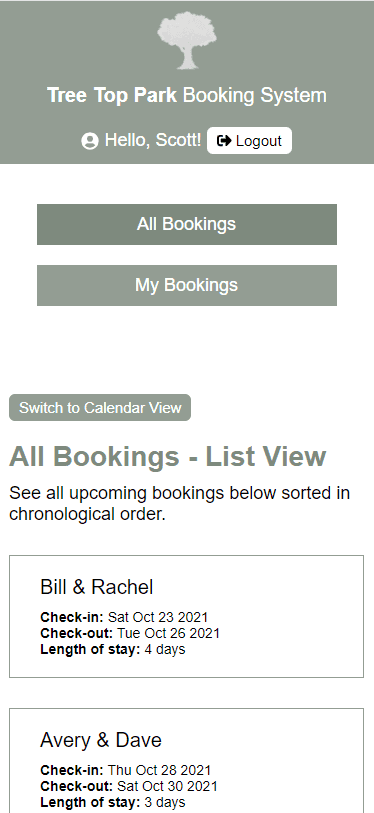The image is a portrait-mode screenshot of a booking system interface for "Treetop Park". The top section features an olive green background with an outline of a fluffy tree, likely an oak tree. Below the tree graphic, the title "Treetop Park Booking System" is displayed. Underneath this title, there is a person icon followed by the text "Hello Scott". Adjacent to it, there is a white button labeled "Log Out".

Following this section, a white horizontal stripe divides the screen. Below the stripe is an olive green button labeled "All Bookings". Another white stripe follows, below which there is an olive green button labeled "My Bookings".

The interface continues with a large white section that features an olive green button labeled "Switch to Calendar View". This is followed by a header in olive green text reading "All Bookings List View". Below this header, the text "See all upcoming bookings below sorted in chronological order" is displayed.

The main content area contains a series of bordered rectangles listing booking details. The first rectangle displays:

- Names: Bill and Rachel
- Check-in: Saturday, October 23, 2021
- Check-out: Tuesday, October 26, 2021
- Length of stay: 4 days

A white stripe separates this booking from the next. The second rectangle shows:

- Names: Avery and Dave
- Check-in: Thursday, October 8, 2021
- Check-out: Saturday, October 30, 2021
- Length of stay: 3 days

In each booking rectangle, the terms "Check-in", "Check-out", and "Length of Stay" are in bold text, highlighting these key details. The entire screenshot depicts a system interface used for managing rental bookings at Treetop Park.